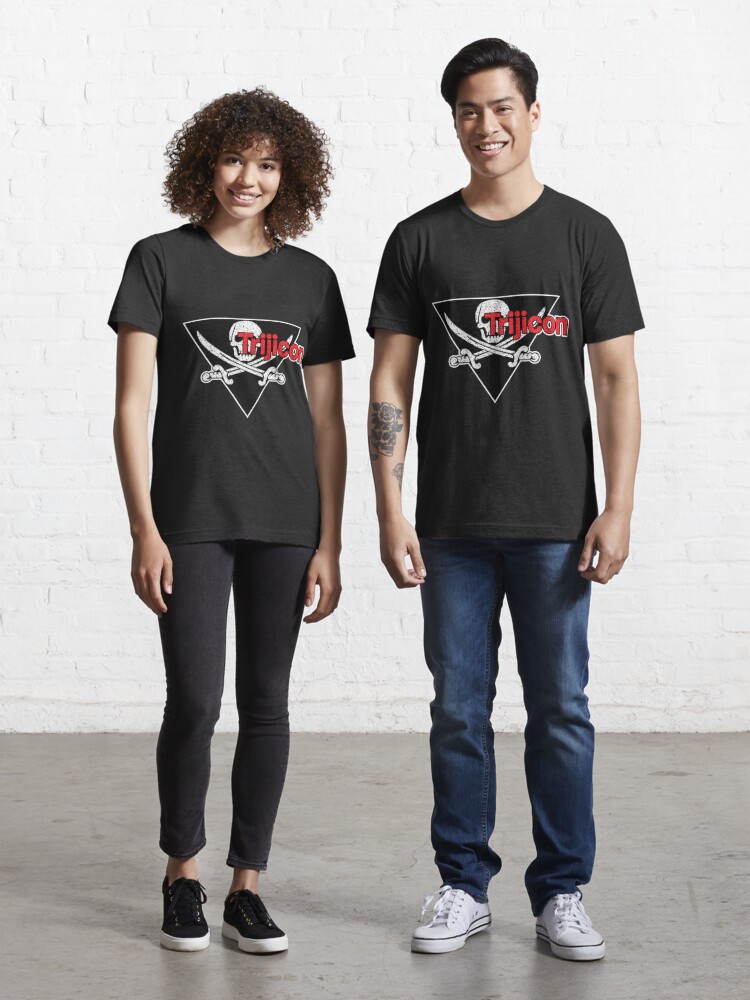In the photograph, two people stand in the center of a room, smiling warmly at the camera. The room features a grey floor and a white brick wall in the background. Both individuals, a woman on the left and a man on the right, are dressed in similar black t-shirts adorned with a distinct triangular logo. The logo is white and prominently features a skull with two crossing swords beneath it, accompanied by red text that reads "TRIGICON." 

The woman, who appears to be either Latina or of mixed black and white heritage, has curly hair and complements her black t-shirt with black trousers and black shoes that have a white base. The man, who seems to be of Asian descent, pairs his matching t-shirt with blue jeans and white sneakers. He also has a visible tattoo on his arm, adding to his stylish appearance. The overall setting and attire suggest a fashion or apparel advertisement, showcasing these coordinated t-shirts with their edgy, eye-catching design.